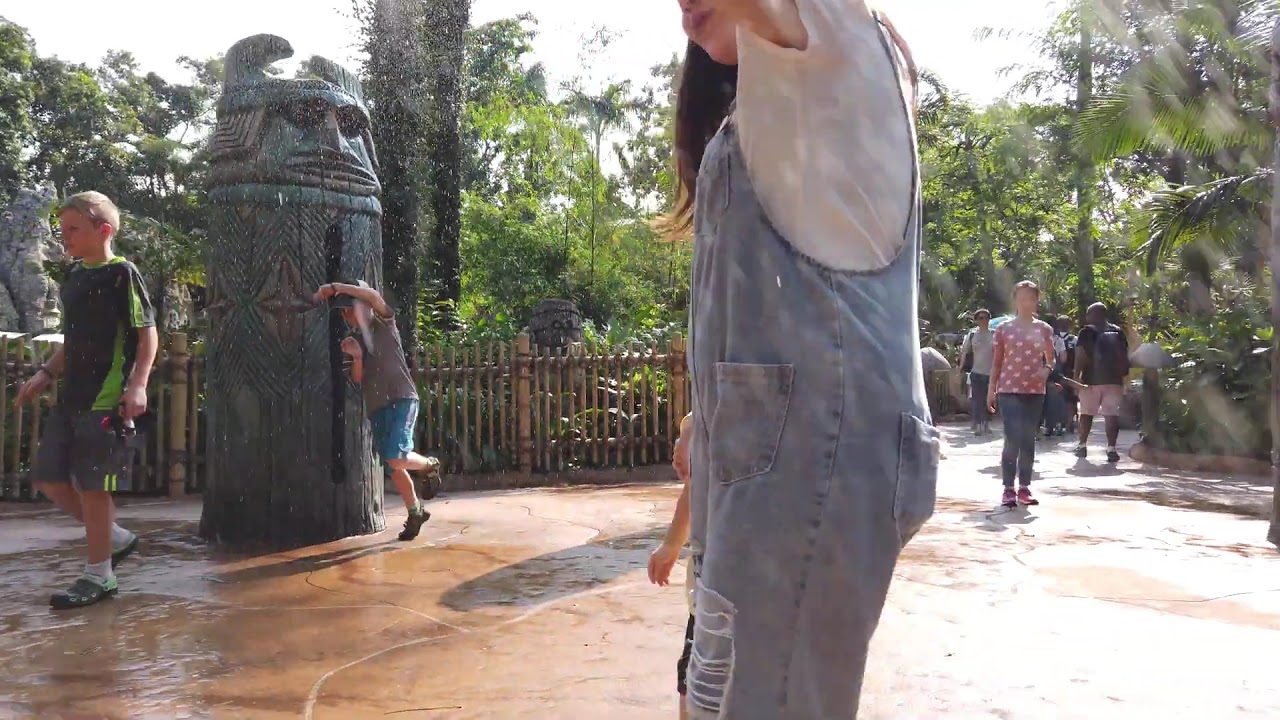In the image, several children are playing outside in a plaza area paved with tannish brown concrete. The focal point is a little girl, who occupies the center of the image, though the top of her face is cut off from her nose upwards down to her knees. She faces left and is dressed in blue jean overalls with a short-sleeve white shirt, her left arm pointing skyward. She has long brown hair. Behind her, to the left, is a large, dark gray, totem-like wooden statue with a water feature, and under the statue, a little boy stands wearing a brown shirt and blue shorts. Another child, to the far left, wears a green and black shirt, gray shorts, and crocs with socks. The setting includes some fencing on the left and a walkway with pedestrians on the right, bordered by lush greenery and some palm trees in the background.